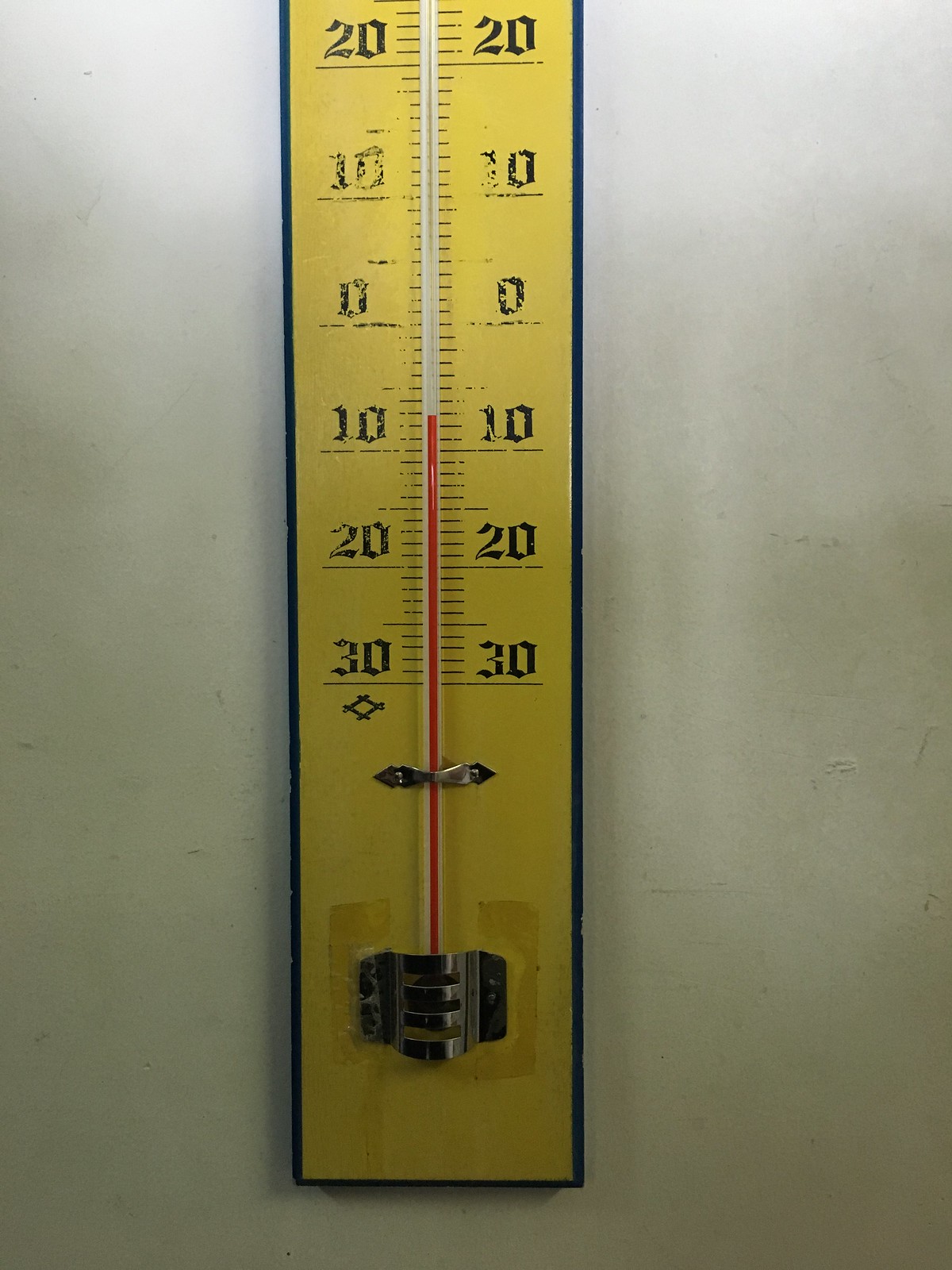The photograph captures an indoor setting, featuring a white wall adorned with a yellow thermometer. The thermometer has a sleek black border and dual rows of numerical markings running parallel to each other. These numbers, in descending order, read 30, 20, 10, 0, 10, 20, and 30.

A slim glass tube containing red mercury runs vertically along the thermometer, with the mercury level slightly above the first '10' mark, indicating a temperature between 10 and 20 degrees. Each number is accompanied by small outward ticks for precise readings.

The thermometer is secured to the wall with two silver brackets: a small one near the middle holding the mercury tube, and a larger one at the bottom providing additional support. There is a slight discoloration, possibly residual glue, near the bottom bracket, marring the otherwise consistent yellow paint of the thermometer.